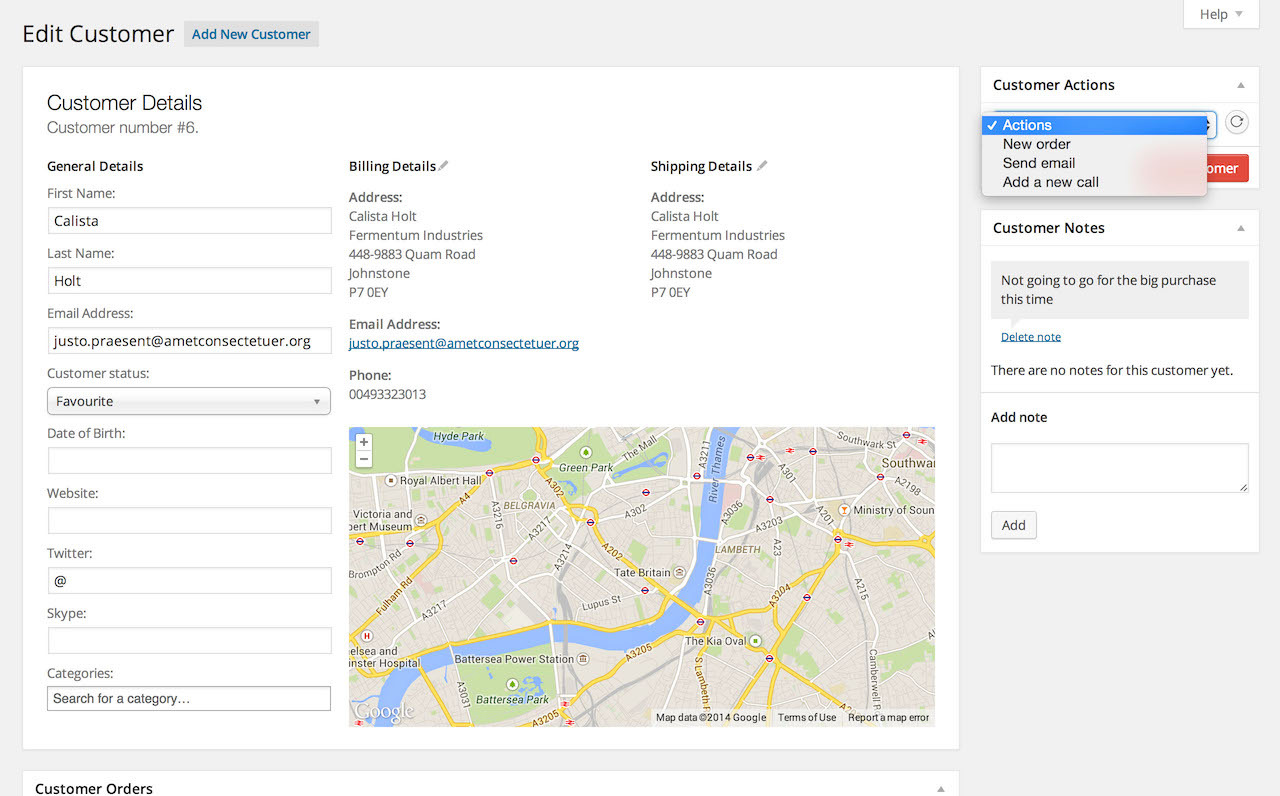In the upper left corner of the interface, there's a section labeled "Edit Customer," accompanied by a gray button with blue text that says "Add New Customer." The background of the entire interface is gray. On the right-hand side, there is a help button in a lighter gray shade that unveils a dropdown menu when clicked.

Dominating the center of the interface is a large, horizontally-oriented white rectangle. In the top section of this rectangle, "Customer Details" is prominently displayed in black font. This section includes various fields, such as the customer number (6), general details, and specific information about the customer. The first name is "Calista," the last name is "Holt," and the email address is "justo.praesent@metcourt.org." Additional details include the customer status, listed as "Favorite," and fields for the date of birth, websites, Twitter, and Skype, all of which are currently blank. Below these fields, there is an option to "Search for Categories."

On the right side of the same rectangle, a subsection titled "Billing Details" provides further information: "Castelia Holt" of "Fermentum Industries," residing at "448-9883 Quam Road, Johnstone, P7OEY." Beneath these billing details, a map is displayed, offering a visual representation of the location.